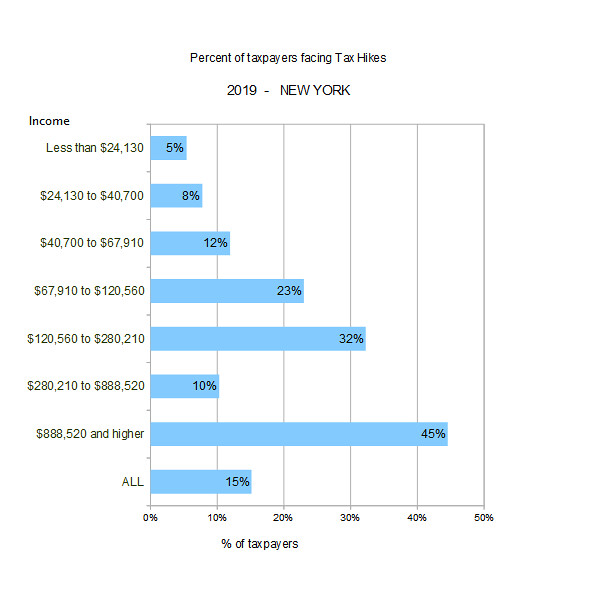The bar chart, titled "Percent of Taxpayers Facing Tax Hikes, 2019 - New York," displays the percentage of taxpayers impacted by tax increases, segmented by various income levels. The text is prominently in green, with black lines delineating different sections, and blue bars representing the data. Each bar features both numerical and percentage values. The income ranges listed on the left include: less than $24,130 at 5%, $24,130 to $40,700 at 8%, $40,700 to $67,910 at 12%, $67,910 to $120,560 at 23%, $120,560 to $280,210 at 32%, $280,210 to $888,520 at 10%, and $888,520 or higher at 45%. The overall percentage of taxpayers facing tax hikes is noted at the bottom, measuring 15%. The chart’s axis at the bottom indicates a percentage range from 0% to 50%.